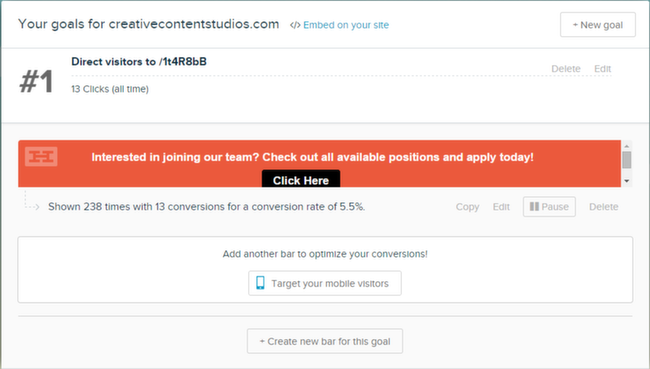Sure, here's a detailed and cleaned-up caption for the image:

---

The image depicts an interface from Creative Content Studios' website, showcasing their goals directive feature. The page includes several elements designed to help users manage and embed goals into their sites. 

1. **Header and Navigation**:
   - The top section features a **large “H” logo** located in the upper left corner on an **orange background**.
   - In the upper right corner, there is a button with a **plus sign labeled "New Goal"**.

2. **Main Goal Section**:
   - The primary goal is indicated by a **large pound sign followed by the number one**.
   - The goal, labeled **“Direct visitors to /1T4R8BB”**, which has had **13 clicks all-time**. 
   - Below this, there are options to **delete** and **edit** the goal.

3. **Embedded Text Field**:
   - There is a distinct **orange field** that prompts: **“Interested in joining our team? Check out the available positions and apply today, click here.”**
   - It shows data indicating that the prompt has been displayed **238 times with 13 conversions**, yielding a **conversion rate of 5.5%**.
   - Next to this information, there are options to **copy**, **edit**, **pause**, or **delete** the prompt.

4. **Additional Features**:
   - Beneath the main goal section are prompts to **"Add another bar to optimize your conversions,"** including a suggestion to target **mobile visitors** with a cell phone icon.
   - Lastly, there is an option to **“Create new bar for this goal”**.

This efficient user interface helps users to seamlessly manage their goals, track performance metrics, and optimize conversions.